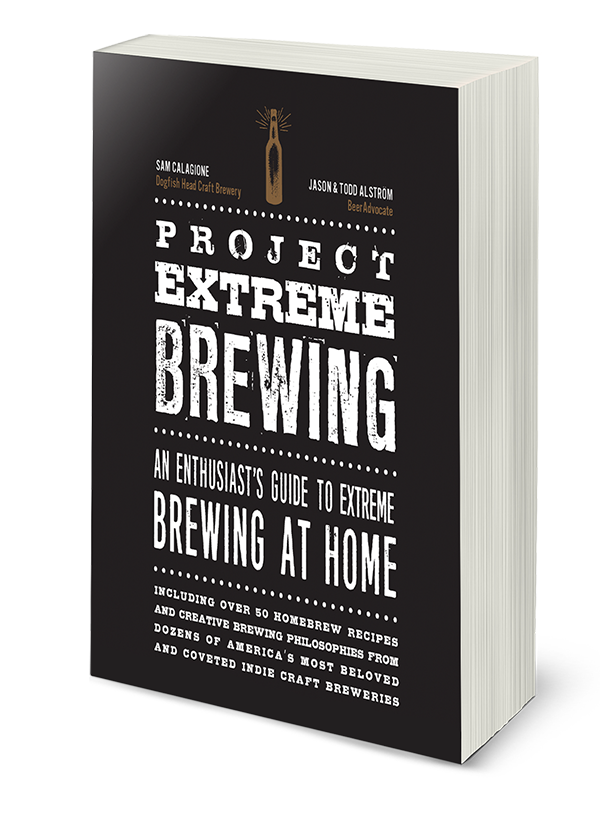This is an image of a black book cover titled "Project Extreme Brewing: An Enthusiast's Guide to Extreme Brewing at Home." The cover features white typography and a small brown image of a bottle at the top. The subtitle notes that the book includes over 50 homebrew recipes and creative brewing philosophies from dozens of America's most beloved and coveted indie craft brewers. The book appears to be about 300 pages long. Authored by Sam Calagione along with Jason and Todd Alström, this guide is a comprehensive resource for homebrewing enthusiasts. The names of the authors are positioned near the top left corner, adjacent to the small bottle image.